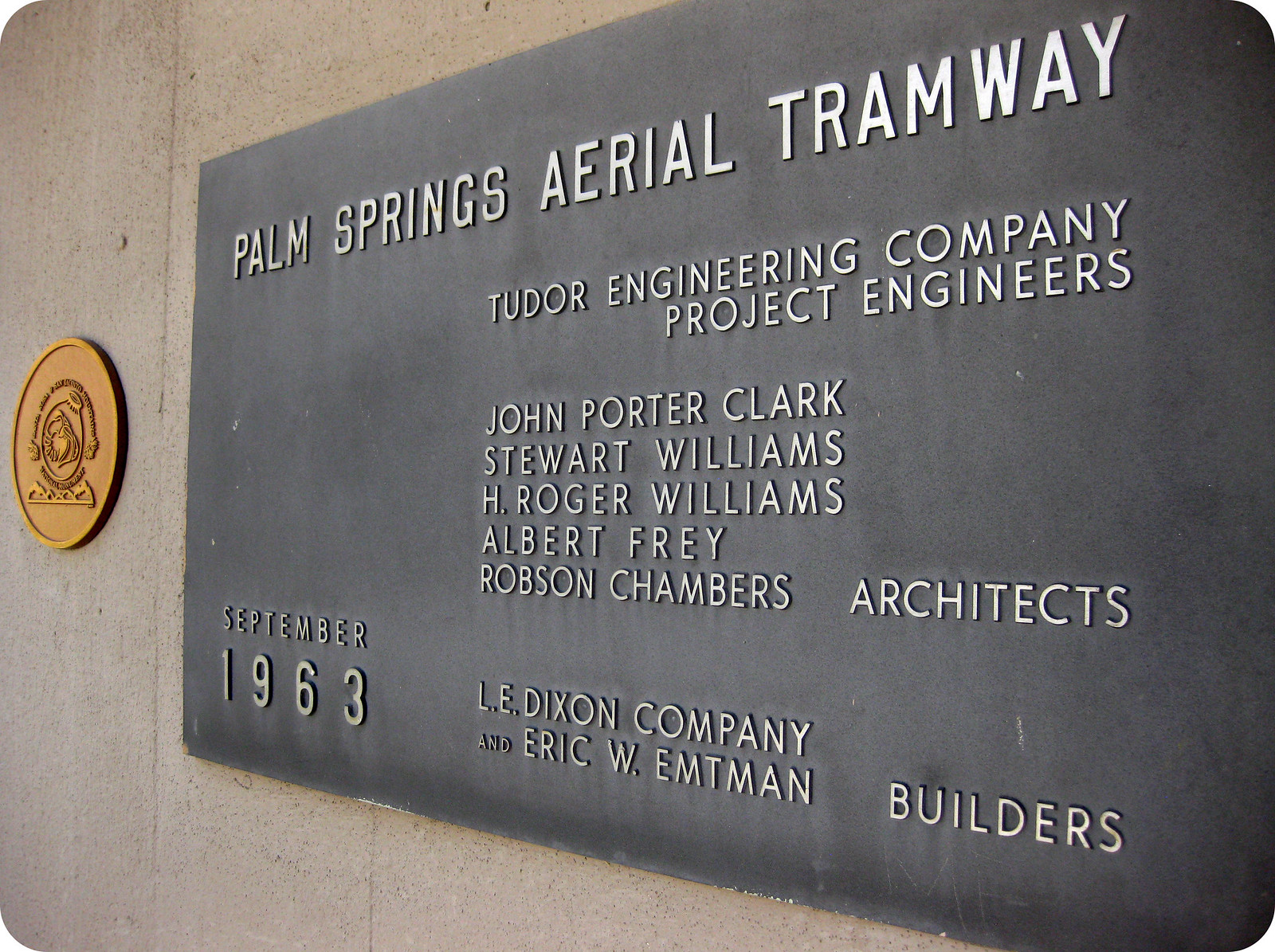The photograph depicts a large, light gray plaque mounted on the beige stone exterior of a substantial building. Captured from a diagonal perspective, the rectangular plaque features white, capitalized text against a black background. It prominently displays "Palm Springs Aerial Tramway" followed by "Tudor Engineering Company, Project Engineers." Below this, the plaque lists the team members: John Porter Clark, Stuart Williams, H. Roger Williams, Albert Frey, and Robson Chambers Architects. Further details include the inscription "September 1963," "L.E. Dixon Company," and "Eric W. Empman Builders." Adjacent to this main plaque, on the right side, there is a smaller, circular plaque in a coppery gold color with text and an intricate emblem that appears to depict mountains and a heart-like symbol surrounded by additional text.